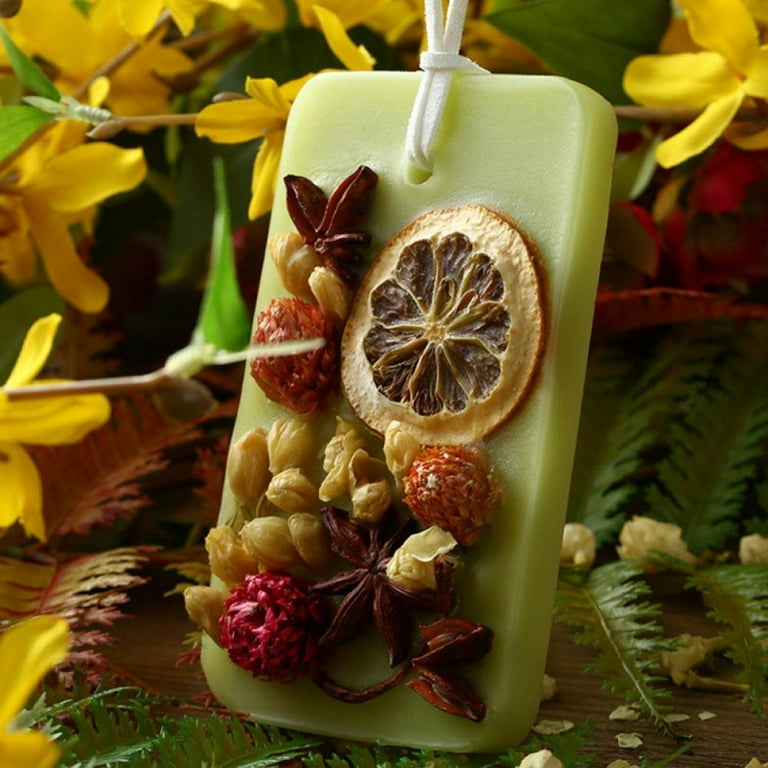The image showcases a meticulously crafted object, prominently featured in the center of the frame. This object is a light green, rectangular slab resembling a bar of wax or soap. It has a distinctive hole at the top threaded with a white string, suggesting it might be hung as a decorative piece. Embedded within the surface of this lime-green slab are an assortment of dried elements: a prominent dried orange slice, raspberries, cloves, pumpkin seeds, and various colorful dried flowers in shades of pink, orange, light yellow, and deep purplish-red, giving it a rustic, artisanal appearance.

The slab is set on a wooden table, with the rich brown tones adding warmth to the scene. Surrounding the table is a vibrant arrangement of green and red ferns, accentuated by yellow flowers that frame the composition beautifully. The background is slightly blurred, enhancing the depth of the image and focusing attention on the central object. The autumnal hues of the leaves and flowers provide a seasonal context, creating a cozy, inviting atmosphere. The combination of natural elements and crafted art in this photograph exudes charm and detail, making it visually engaging and richly textured.